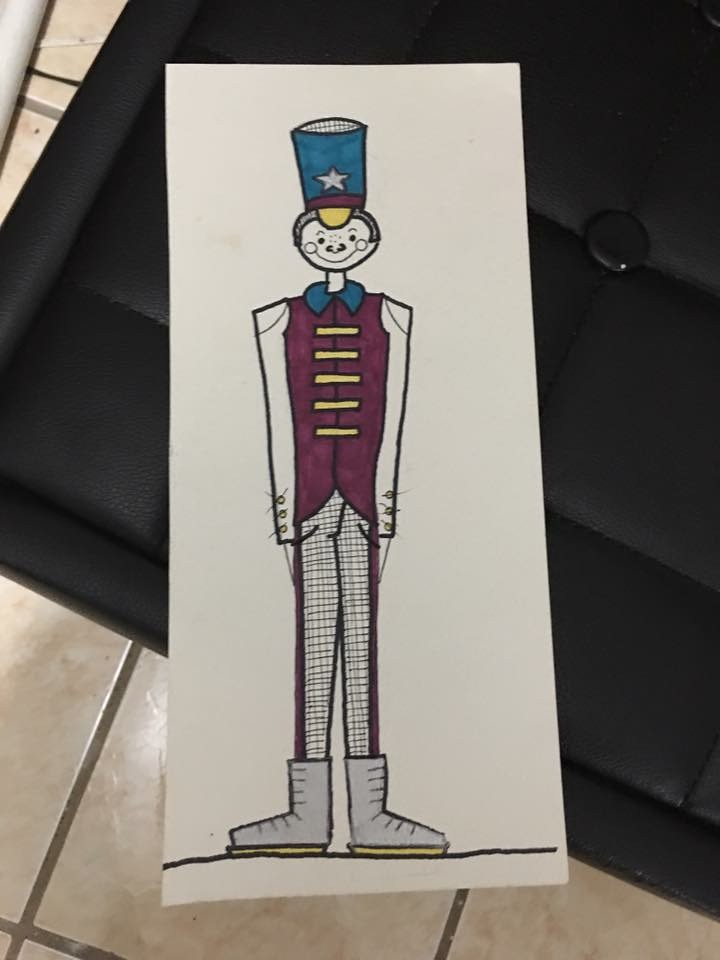The illustration appears to be a whimsical, cartoonish representation of a toy soldier or possibly an ice skater, drawn on a narrow, rectangular piece of white paper. The figure is adorned in a highly detailed and colorful outfit reminiscent of a marching band uniform. This ensemble includes a vibrant purple vest with four horizontal yellow bars, complementing the turquoise blue collar. The sleeves extending from underneath the vest look white, adding to the overall brightness of the outfit. The pants are striking with a black and white checkered pattern, each leg adorned with a purple stripe down the side. The figure's feet are clad in gray boots, each featuring a yellow band at the bottom that resembles ice skate blades.

The character also sports a tall, eye-catching turquoise hat embellished with a bright blue star and accented with both a yellow brim and a purple and yellow visor. The face is rendered in a circular, cartoon style with prominent round cheeks, a large smile, and small eyes, all topped with what appears to be short black hair.

This drawing is placed on a black leather surface, likely an ottoman or the edge of a couch, and partially hangs off its support. Beneath the illustration, a beige, square-tile floor is visible, adding a textured backdrop to the scene.